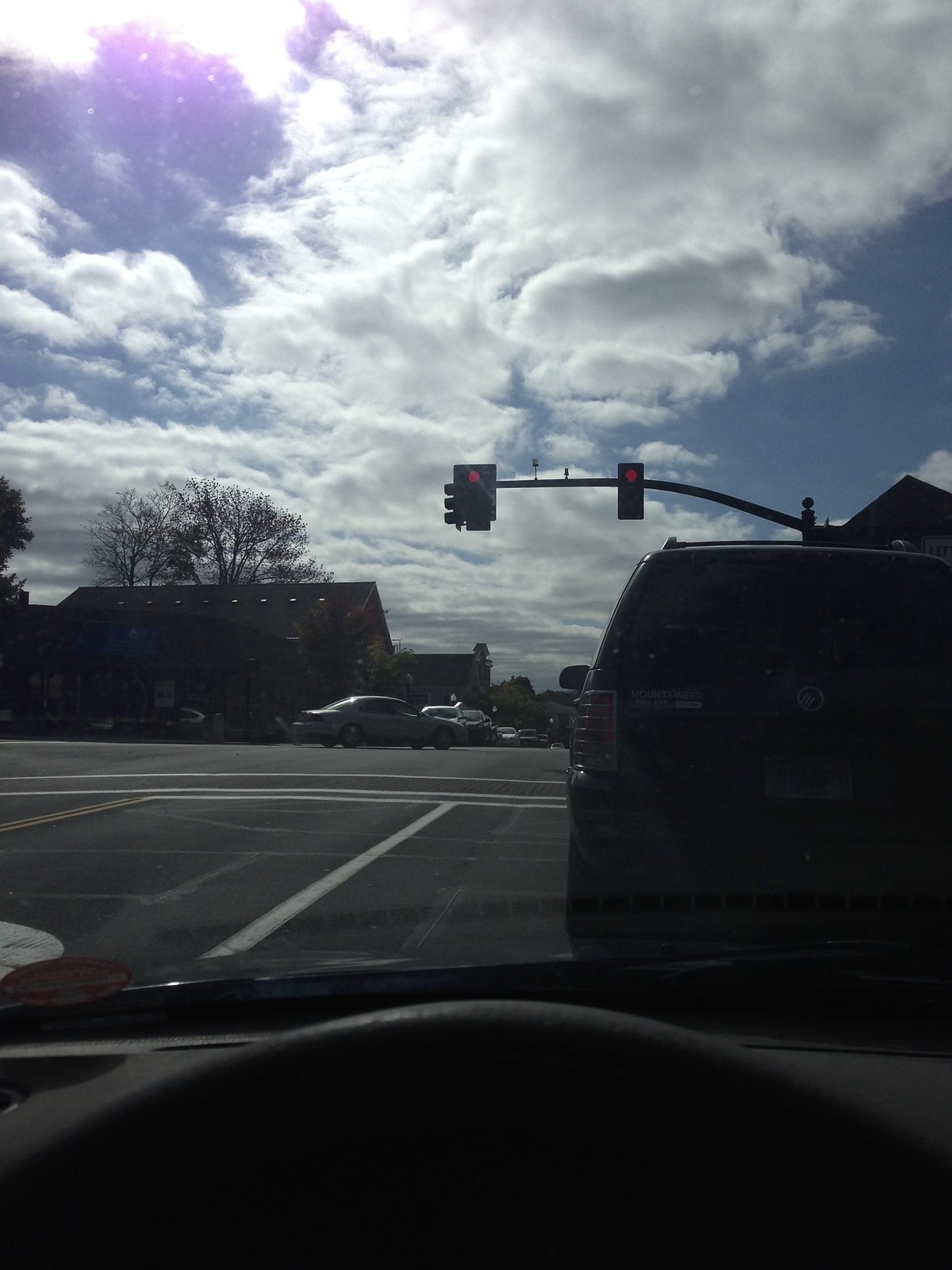The image captures a scene from inside a parked or stopped car at a red traffic light. The photo, taken from the driver's perspective, includes the dark steering wheel and dashboard, contributing to the overall dim tone of the interior despite the daylight outside. Directly in front of the car is a large black SUV, also waiting at the light. Beyond the intersection, other cars are visible, including a white car driving across and a gray vehicle in the middle of the intersection attempting a left turn. Surrounding the scene are various houses and buildings, likely businesses, with a small leafless tree noted on one corner. Puffy white clouds scatter across a blue sky with the sun shining through, though partially cut off at the top left-hand side of the image. The car’s windshield features a circular red sticker at the bottom left, while the SUV ahead bears a sticker near its brake light.